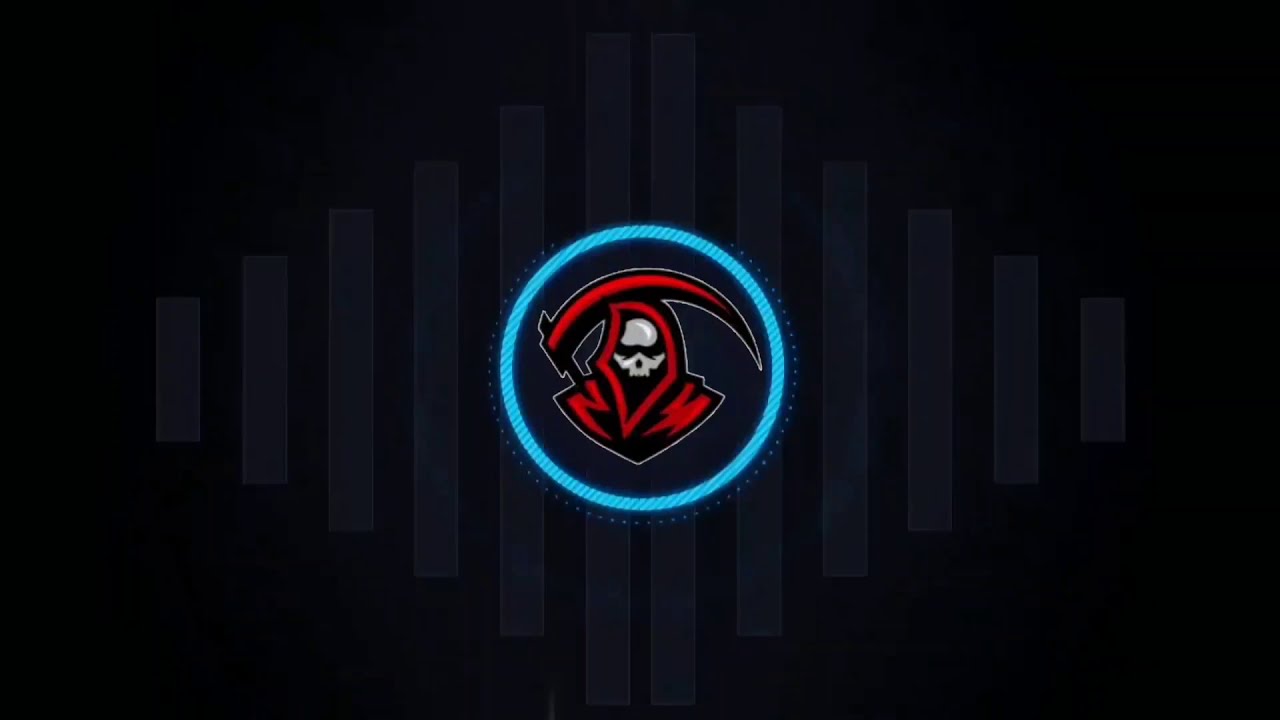The image depicts a high-definition, horizontally-oriented digital photo featuring a dark and somewhat black background with dark gray vertical stripes that stretch longer as they approach the center, resembling Wi-Fi bars or signal indicators. Central to the image is a glowing neon blue circle outlined in bright fluorescent blue, filled with smaller glowing blue dots emanating around it. Within this circle sits a vivid red Grim Reaper emblem, showcasing a white skull face under the hood, but no visible body below the shoulders. Behind the Reaper, a red scythe arches across, adding to its ominous appearance. The design strongly promotes the central figure, drawing the viewer’s attention with its luminescent qualities against the darker backdrop.